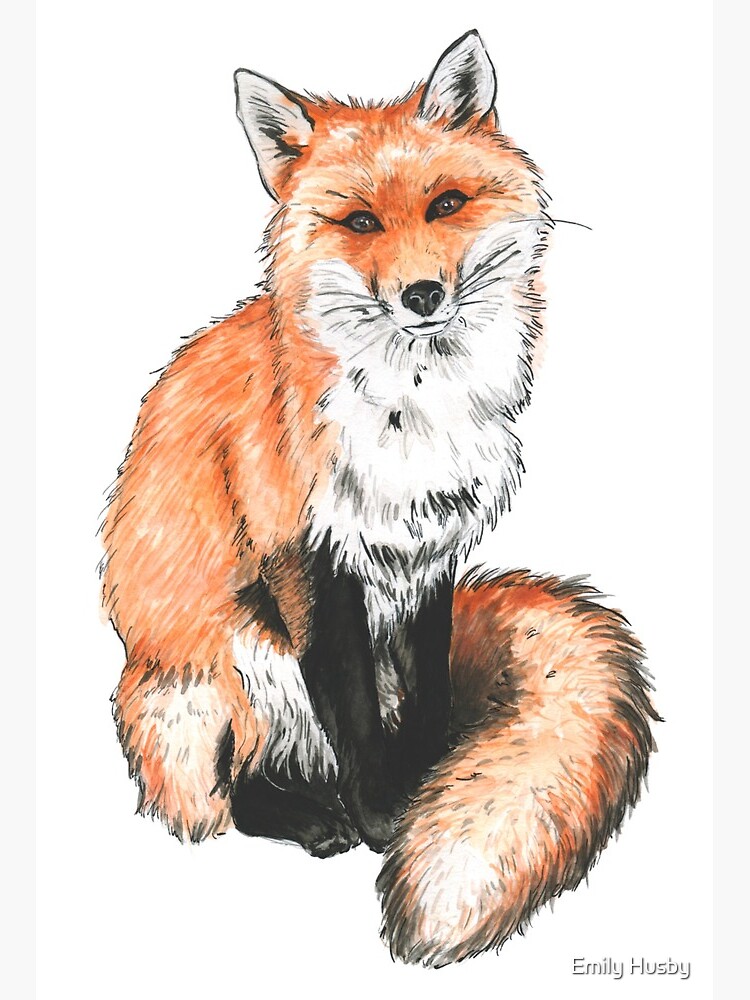This is a highly detailed sketch of a fox by Emily Husby, whose name is signed in the bottom right corner in white bubble letters with a black shadow. The sketch showcases a fox sitting with its tail curled around its legs. The fox's head is slightly cocked to the right, and it gazes directly at the viewer with a happy expression and bright, reflective brown eyes. The illustration uses a reddish-orange hue for the fur, with several shades of orange for depth, while the chest and parts of the ears are white. The fox has a black nose, long whiskers, and black fur on its feet and arms. The ears are outlined in black and are perked up. The sketch employs a rough style with light strokes and darker lines to highlight the arms, fur, and borders, giving it a very lifelike appearance.